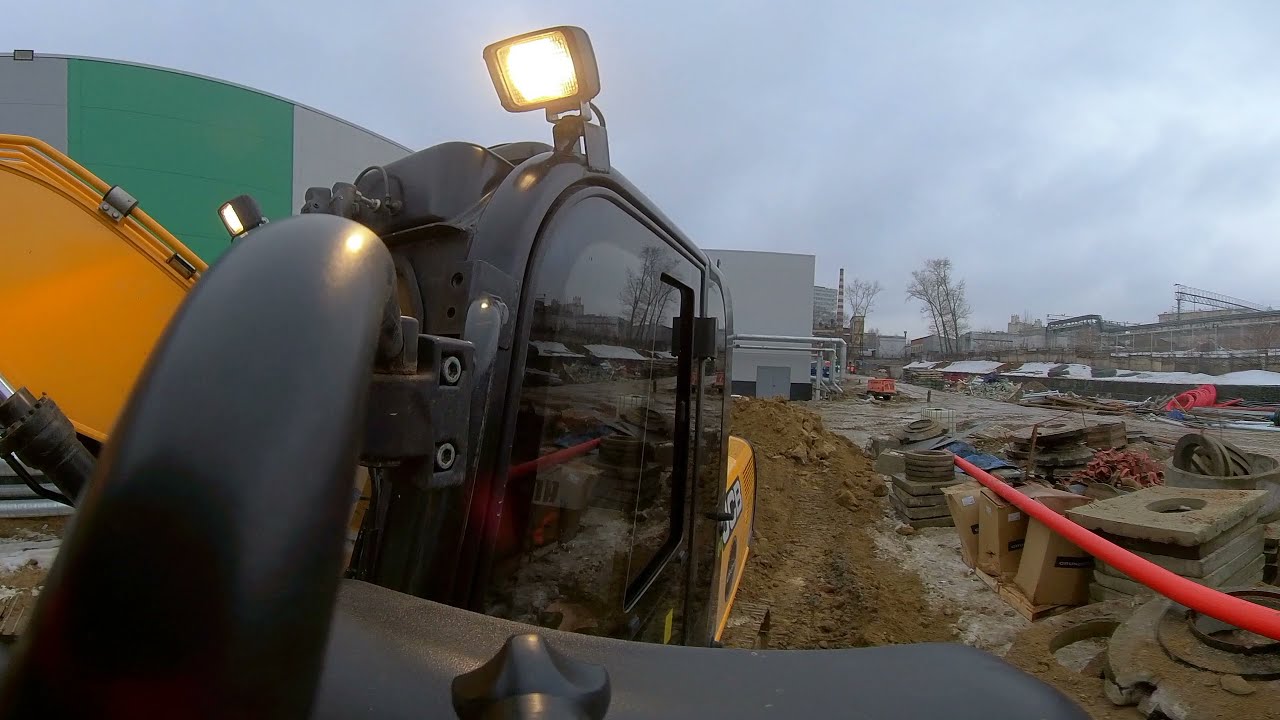The image, taken during the daytime at a construction site, prominently features a piece of construction equipment, likely an excavation tractor, with a mounted camera capturing the scene. The cabin of the tractor is visible with a large window door and a partially seen bright yellowish-orange arm, suggesting it might be a crane vehicle. The cabin itself is framed in black, featuring squared lights that emit an amber glow. The tractor is placed on disturbed brown dirt, which covers much of the site.

On the tractor's left side, there is a notable heavy machinery component with a light. The middle right of the image showcases various construction materials, including slabs of concrete and boxes. Adjacent to these materials, you can identify planks of wood and a red and orange hose against a barrier.

In the backdrop, a large industrial building dominates with its grey facade, marked by a distinct green stripe running vertically. To its left, another grey warehouse-like structure is visible, adding to the industrial atmosphere that recalls areas like the still-industrial parts of Detroit. The entire scene is framed by the gritty textures and rugged elements typical of an active construction site.